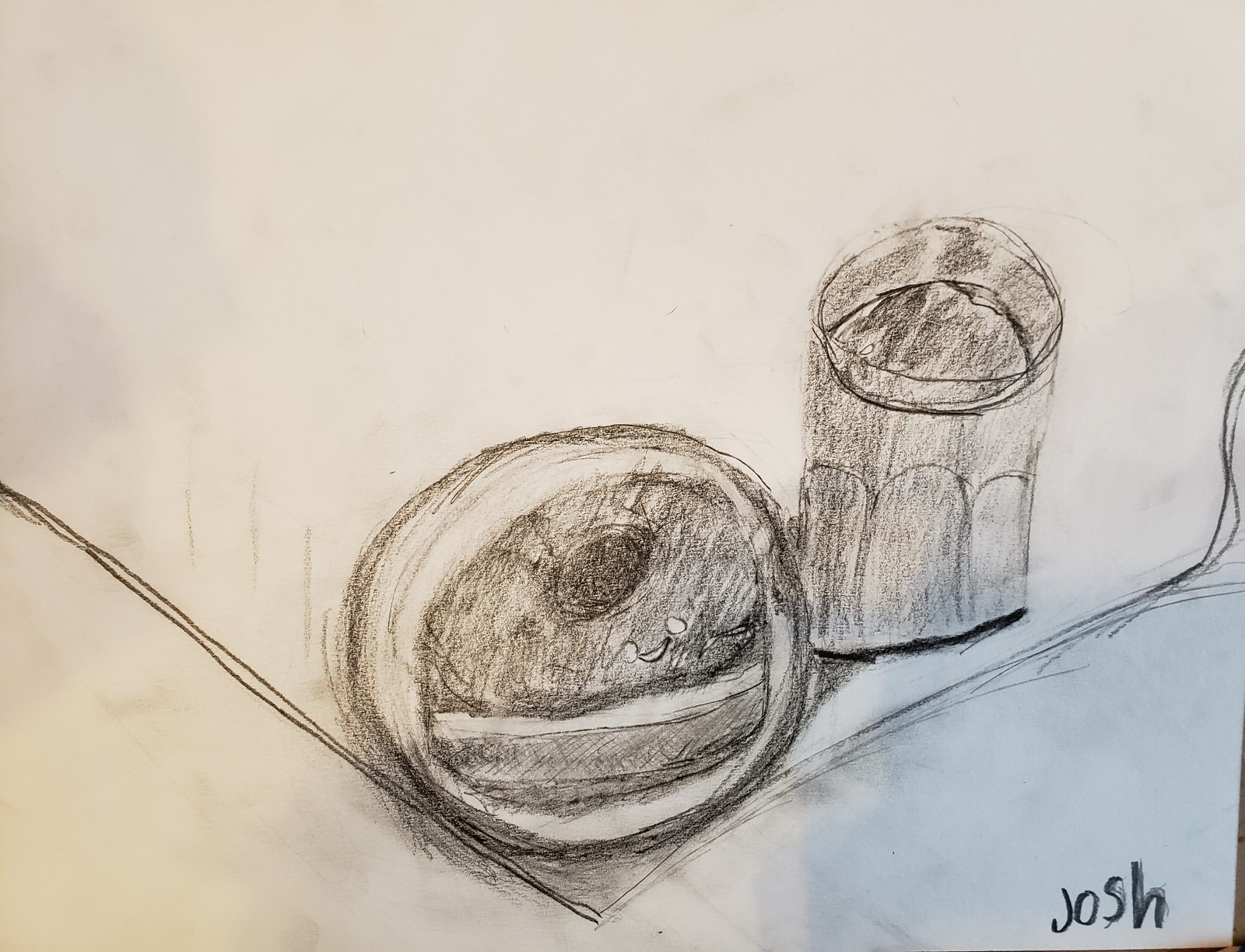This is a detailed, hand-drawn pencil sketch on what appears to be faded tan drawing paper. The drawing prominently features a circular object in the center, which resembles a bagel sandwich or perhaps a doughnut on a plate. This circular object has a dark, shaded bottom part, a white layer in the middle, and a lightly shaded top part with a hole in it. To the right of this object, there is a small drinking glass with varying degrees of shading. Additionally, in the upper right area of the image, there appears to be a depiction of a sugar or salt shaker. The lower portion of the image includes diagonal lines creating a sense of depth and structure. In the bottom right corner, the artist's name, "Josh," is clearly signed, indicating the creator of this meticulously shaded artwork.